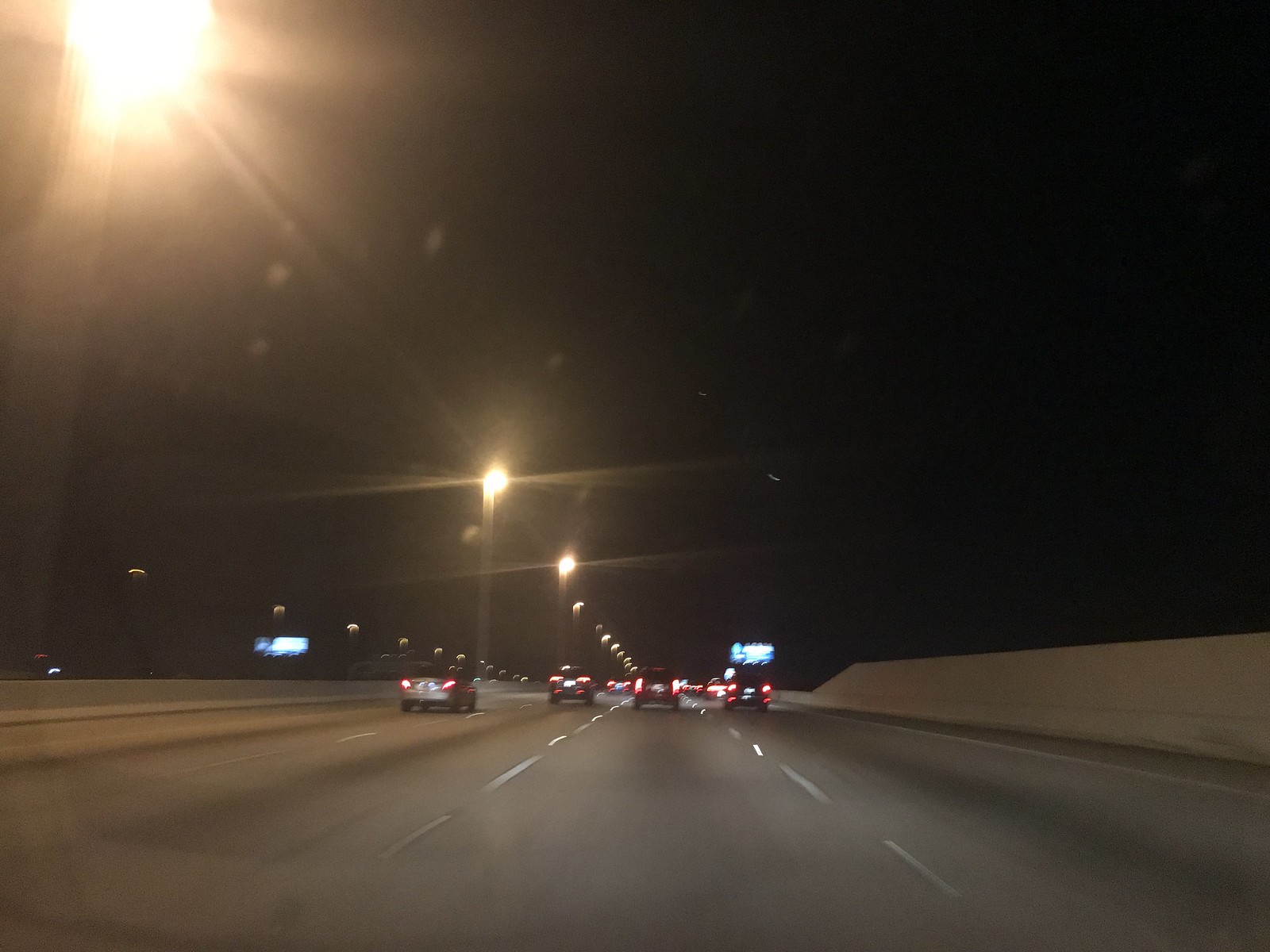The image captures a nighttime scene of a multi-lane highway viewed from an elevated vantage point, possibly a bridge. The roadway extends into the horizon, with four lanes moving away from the viewer. To the left side of the image, the opposite-direction lanes are slightly visible. The highway features a low concrete median that becomes taller at the bridge's section. Street lamps, mounted on poles lined along the median, cast pools of light onto the black asphalt, illuminating the surroundings. Two brightly lit billboards appear in the distance, one on either side of the highway, displaying white and blue hues. Vehicles populate all four lanes ahead, highlighted by the street lamps that stretch far into the distance. Additional street lamps are discernible on the outer side of the far lanes, hinting at the opposite traffic. The surface of the road appears to be concrete.